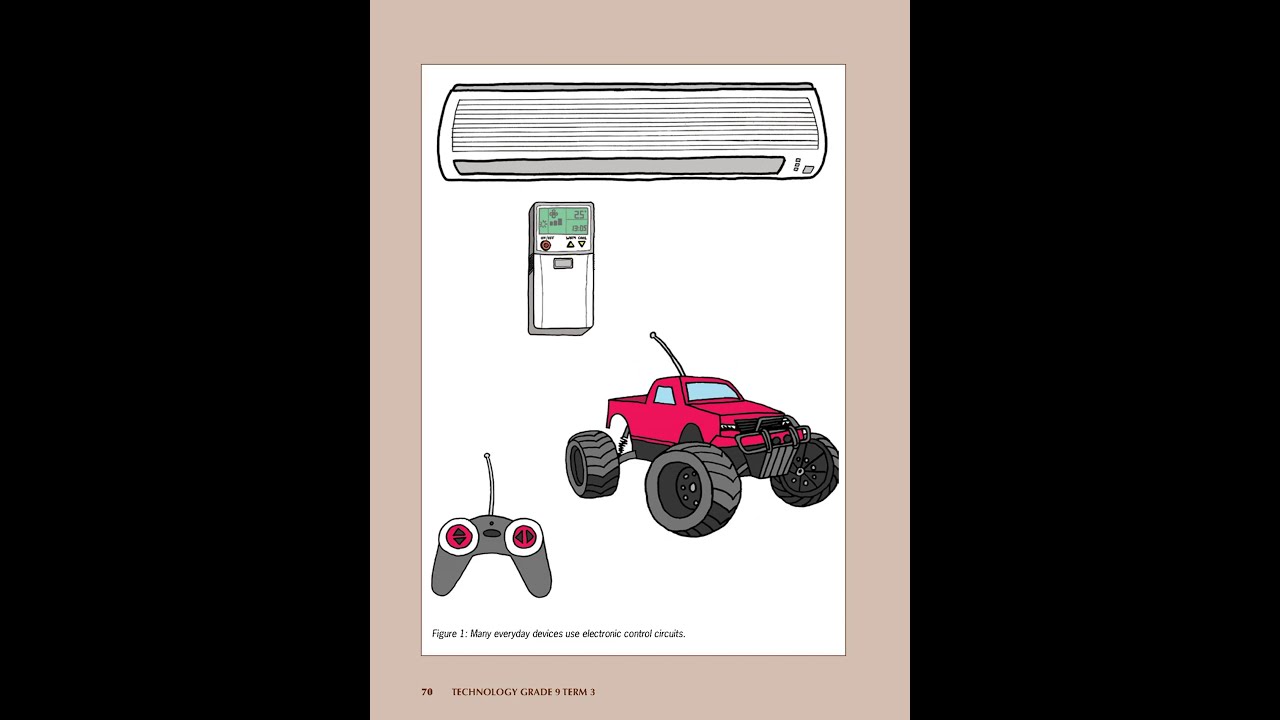This image features a digitally created, colorful drawing set against a solid black background, with a central tan rectangle enclosing various objects. At the top of the tan background is a long horizontal white rectangle with black and white lines, resembling a split air conditioning unit. Beneath this, there's a gray bar whose function is not immediately clear. Below the bar is a vertical white rectangle, simulating a small handheld remote control with a green screen and a few buttons, including a red power button and two arrow buttons. 

The central and most prominent figure in the image is a red monster truck equipped with an antenna and large gray wheels with black trim. To the left of the truck is a gray video game controller, featuring two white circles with red centers and additional control buttons. 

The detailed caption accompanying the image indicates that this could be an illustration from a book, with visible text in the lower left corner stating, "Figure 1: Many everyday devices use electrically controlled circuits." The objects are arranged centrally within the tan rectangle, surrounded by ample black space on either side, contributing to the image’s organized and clean layout. The colors used include black, tan, white, gray, red, and green.